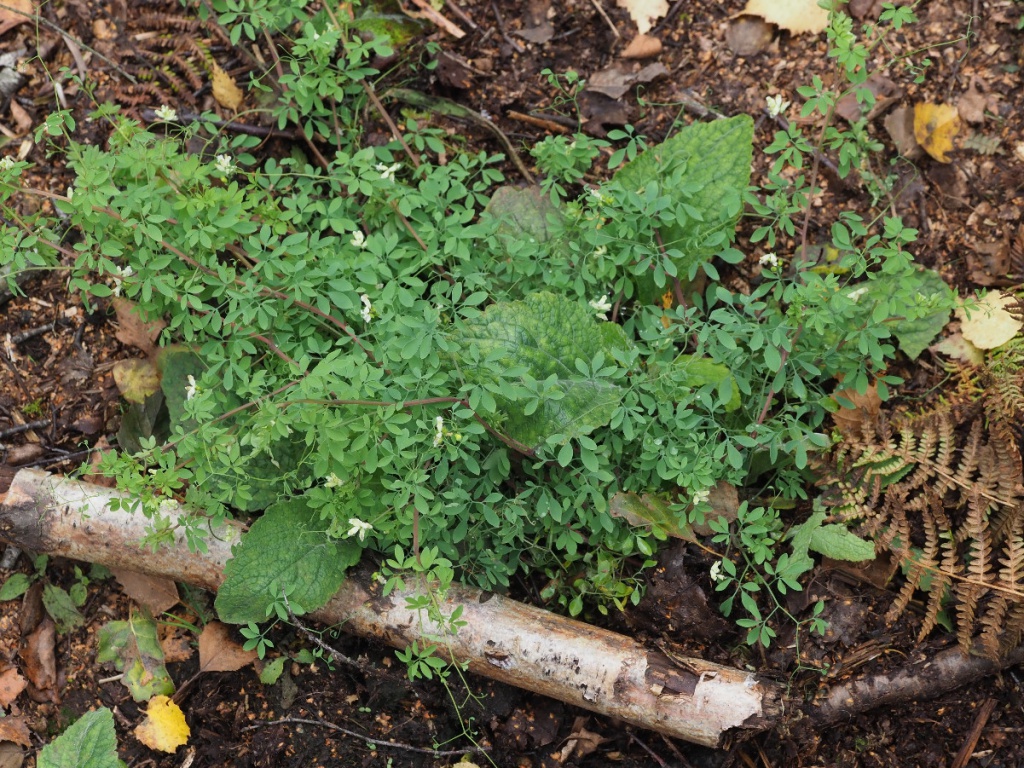The photograph captures an outdoor scene characterized by a muddy, forest-like ground littered with various types of leaf detritus. Central to the image is a dense arrangement of intertwined greenery featuring a mix of tiny leaves with brown stems and larger, diamond-shaped green leaves with slightly rough edges. Among these leaves, small, indistinct white flowers are scattered. A prominent white log lies horizontally in the foreground from left to right, adding to the rustic setting. Surrounding the greenery, there are partially yellowed leaves, brown dead leaves, brown fern litter, and scattered twigs and fallen tree pieces, all laying on the dark brown earth. This striking blend of plant life and woodland debris creates a rich and textured visual of the forest floor.